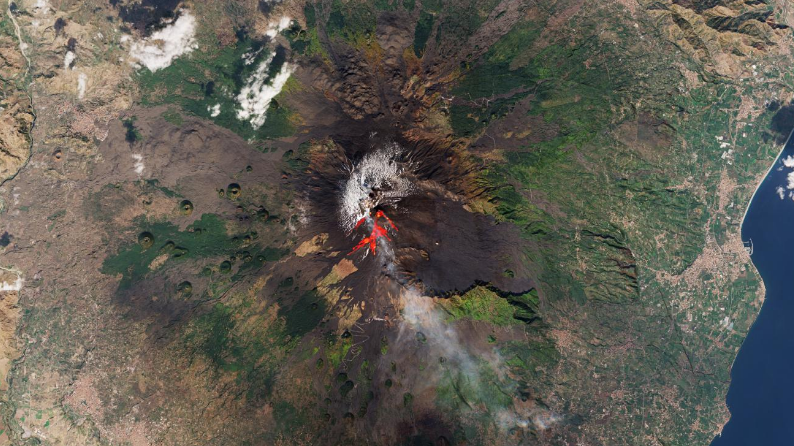The image is an aerial photograph showcasing a somewhat active volcano at its center, characterized by red lava surrounding its top and faint orange hues indicating ongoing activity. The volcano is encircled by large swaths of bare soil and hardened black lava. The land transitions from primarily brown, dry terrain on the left to green, lush areas on the right, suggesting a mixture of uninhabited and vegetated regions. Prominently, white ashes and wisps of smoke rise from the central crater, further emphasizing volcanic activity. On the far right, a body of water is visible, adding a blue accent to the landscape. The overall topography is rugged, with uneven surfaces and rough edges, highlighted by hints of white in the upper sections of the image.